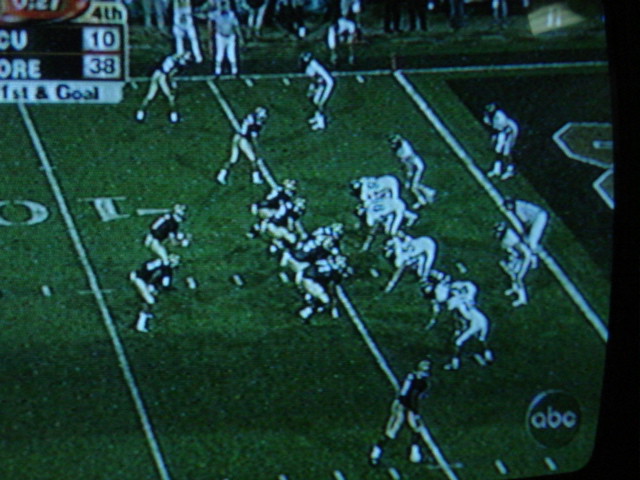The image depicts a television screen broadcasting a football game. The scene shows players lined up before executing a play. The team on the right is wearing white uniforms with black helmets, while the team on the left is outfitted in black shirts, lighter pants, and matching helmets. They are positioned on a green field marked with white lines, near the right-hand side touchdown area. The top of the image includes a portion of the crowd and visible referees. There is a user interface overlay that partially reads "Fourth" along with "CU 10" or "E38" and "First and Goal." The ABC network logo is displayed in the bottom right corner of the screen. The right edge of the TV frame is also visible.